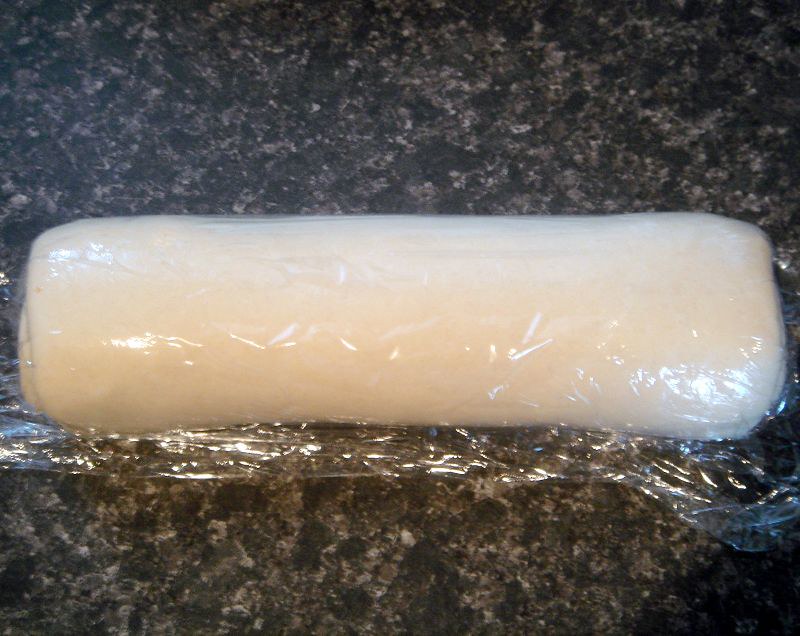This is a close-up image of a countertop that appears to be made of granite, characterized by its mix of grays, including light flecks of nearly white, dark gray, and medium grays, with a dull, non-shiny finish. On top of this countertop is an object wrapped in saran wrap or plastic wrap. The wrapped item is a whitish-beige color and has a smooth, rolled appearance, resembling dough, pie crust, or fondant typically used in cake decorating. The purpose of wrapping it in plastic could be to store it in the fridge or to prepare it for easier cutting into sections. The detailed textures and colors of both the countertop and the wrapped substance create a visually interesting contrast in the scene.